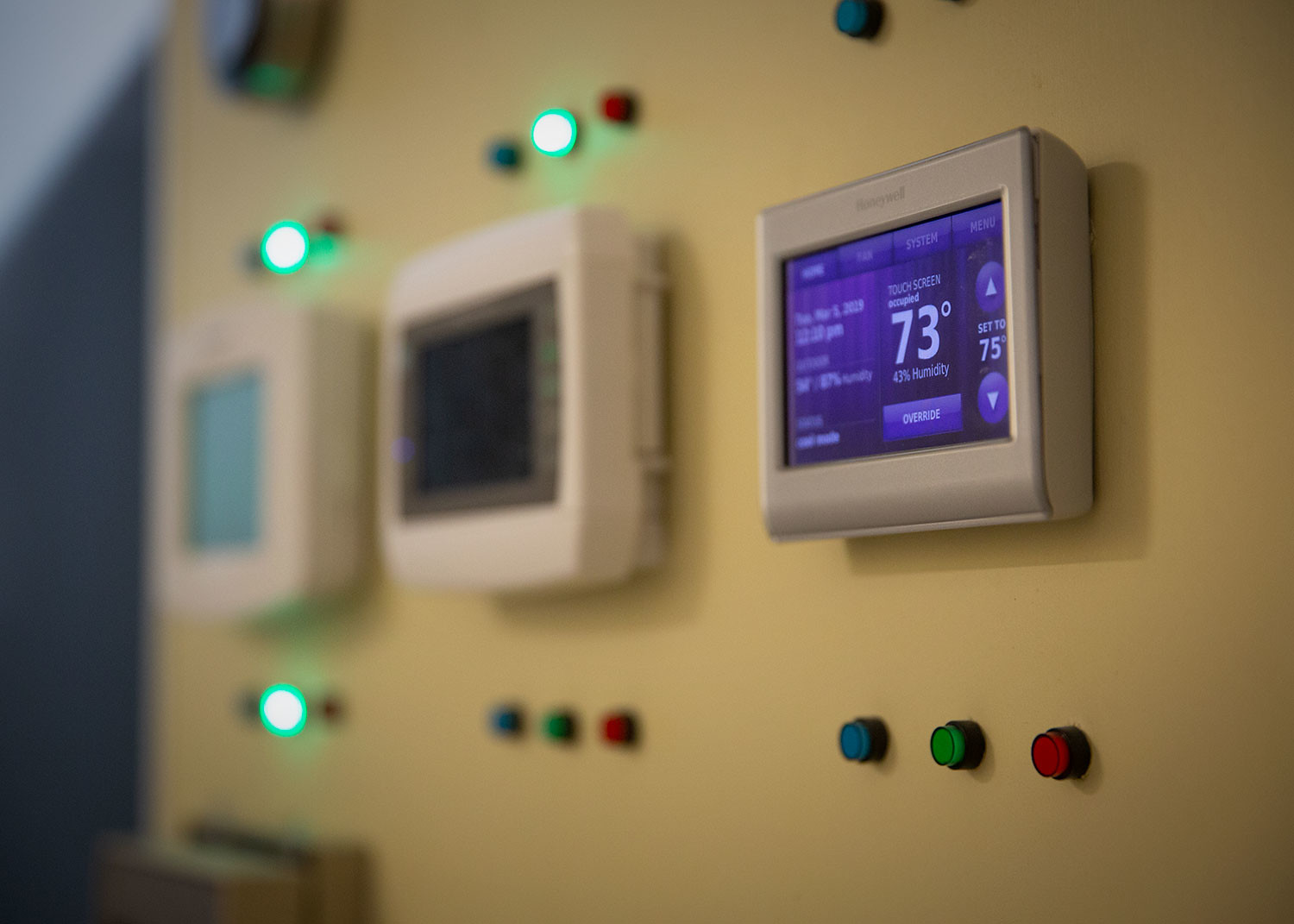The image depicts a yellow wall with three thermostats of varying sizes and presumably from different manufacturers. The overall image is blurry, except for the thermostat on the far right, which is in clear focus. Each thermostat arrangement includes a panel of three indicator lights both above and below the thermostats, colored blue, green, and red from left to right. 

The thermostat on the far left appears to be illuminated, but the blur makes it difficult to discern any details. Both green lights (middle) on the bottom and top panels of this thermostat are visibly lit.

The middle thermostat seems to be off, with no lights illuminated on the bottom panel. However, the top panel shows the green light as lit.

The rightmost thermostat is clearly visible. The bottom row of lights on this thermostat is not illuminated, and the image's cropping obscures the top row except for the blue light. The screen of this thermostat displays various information: it is a touch screen showing a status of "Occupied" with a current temperature of 73 degrees Fahrenheit and 43% humidity. The screen also has menu options, including "System" and "Menu," while the first two options are too blurry to read. The screen indicates that it is Tuesday, March 5th, 2029, and suggests details about the typical temperature or humidity levels. There is a set point of "Set to 75," and a button labeled "Override" alongside up and down toggle arrows.

The presence of these thermostats suggests that temperature control is crucial in this setting, possibly an office or industrial environment where maintaining specific climate conditions is essential.